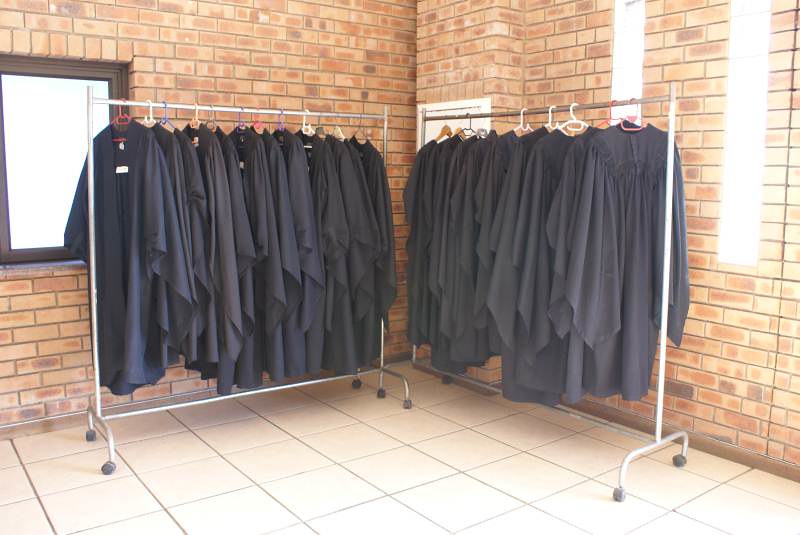This photograph captures a corner of a room with two silver coat racks filled with black robes that resemble graduation or choir gowns. The room features orange-brown brick walls and white square tiles on the floor. On the left side, there's a wooden-framed mirror, while the right side has a white panel with PVC shields. The robes, hanging from colorful plastic coat hangers in red, white, blue, and purple, are neatly arranged, and the racks are mobile, equipped with wheels. A window in one of the brick walls provides a view of the outside.